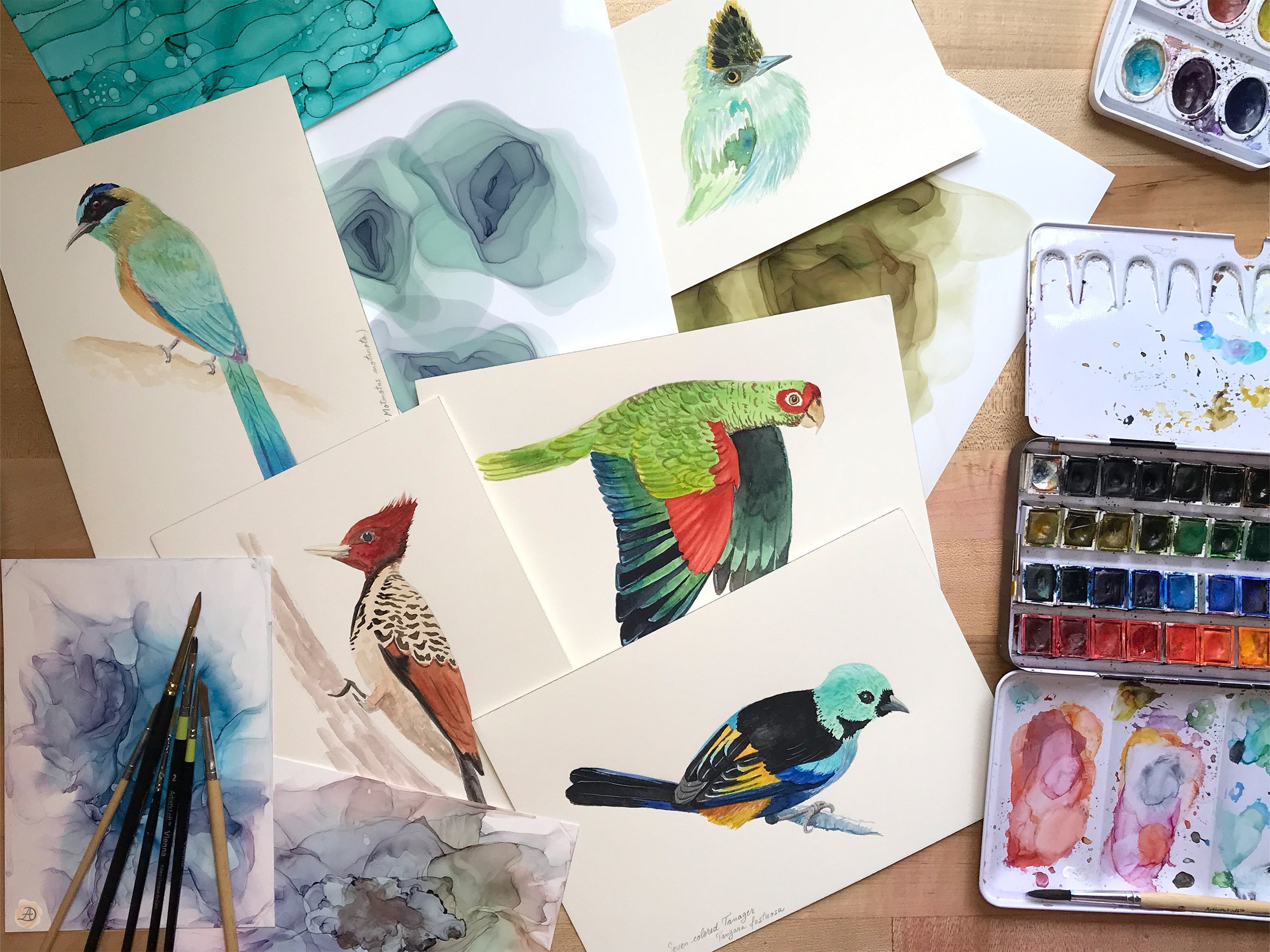This detailed photograph captures the lively workstation of an artist specializing in watercolor paintings of birds. The wooden desk, visible beneath the creative clutter, is covered in a variety of finished and in-progress watercolor images. Spread haphazardly over one another, these vibrant paintings depict a multitude of birds, including a striking parrot in flight, a red-headed woodpecker, and several more exotic and tropical species.

The center right of the image is dominated by two open tins of watercolors, showcasing a rich spectrum of colors from reds, oranges, and browns to blues and greens. These paints, some still wet from recent use, and the lids smeared with blended hues, hint at the artist's dynamic process. Nearby, blotting areas and drying brushes are arranged, indicating constant and varied use.

Among the notable bird illustrations, one features a teal-headed bird with a black eye patch, yellow breast, and blue underbelly, perched elegantly on a branch. Another depicts a woodpecker with a rust-colored head, spotted black and white neck, and a cream underbody, caught in mid-peck at a piece of wood. Yet another vibrant bird displays an array of colors—light green head, red around its eyes, and dark green wingtips.

In addition to the precise bird portraits, there's a smattering of more abstract works and some suggestive forms, including teal gradations resembling underwater scenes and more loosely defined bird-like shapes, adding a layer of experimental creativity to the workspace. Overall, this photograph is a rich tableau showcasing the vibrant and meticulous practice of a dedicated watercolor bird artist.